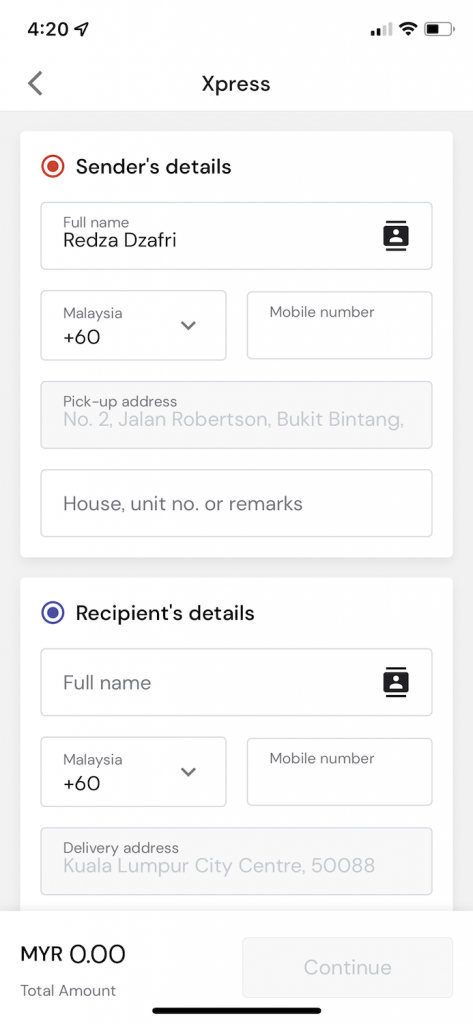In this screenshot, the interface is predominantly white, featuring two main sections: "Sender's Details" and "Recipient's Details". The "Sender's Details" section is identified by a red icon and includes fields for the sender's name, phone number (prefixed by the Malaysian code "+60"), and drop-off address at "2 Jalan Roberts, Bukit Bintang". This section also includes an optional field for house/unit number or additional remarks.

The "Recipient's Details" section, distinguished by a blue icon, requires the recipient's full name, phone number (also prefixed with the Malaysian code "+60"), and the delivery address: "Kuala Lumpur City Central 588". The total amount for the order is displayed as "MYR 0.00", indicating no cost has been calculated yet.

At the bottom, there's a "Continue" button, which is currently inactive, likely due to incomplete information in the required fields.

In the top right corner of the screenshot, the device status bar shows "4:20" and a half-full battery icon. The signal strength appears to be low, as indicated by minimal signal bars.